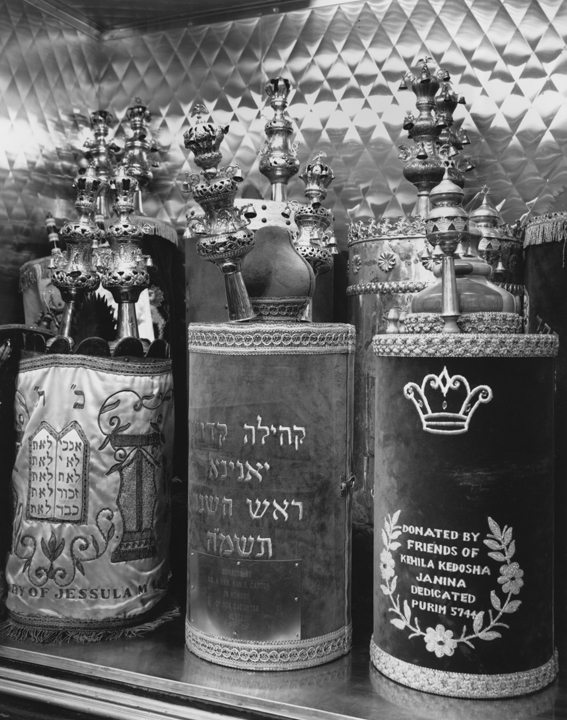The photograph is a color image in portrait orientation, depicting three ornate, cylindrical religious vessels positioned on a chrome base against a diamond-quilted metal background. Each vessel, likely Torah scrolls, is adorned with elaborate tops featuring urn-shaped finials with multiple layers.

The vessel on the left is encased in a fabric cover and displays two tablets with Hebrew writing, possibly representing the Ten Commandments. The central vessel has a different language inscribed on it and also displays intricate decorations. The vessel on the right features a dark background with white Hebrew text that reads, "Donated by friends of Kehillah Kedoshah Janina, dedicated Purim 5744," and is crowned with a detailed finial that includes a wreath motif below the inscription. These items reflect the artistic style of photographic representational realism, capturing the detailed craftsmanship and religious significance of the pieces.